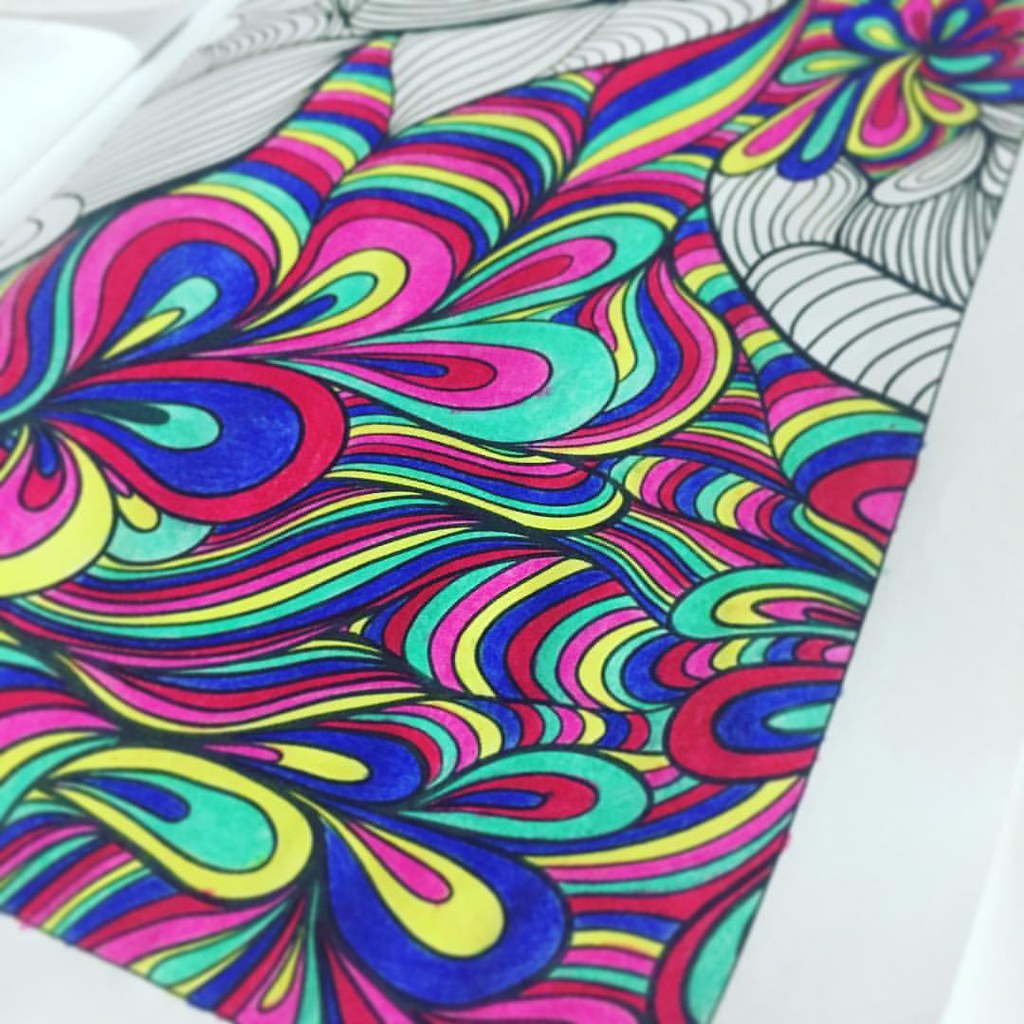A vibrant and intricately detailed page from an adult coloring book is partially colored in with colored pencils. The design features a mesmerizing array of fluid, curvilinear lines that twist and turn in every direction, creating a swirling, psychedelic scene. Shades of blue, yellow, pink, magenta, and turquoise dominate the image, bringing the abstract patterns to life. The page has a clean, white border, and the left side of the image is illuminated by bright sunlight, casting a slight glow on the untouched white space.